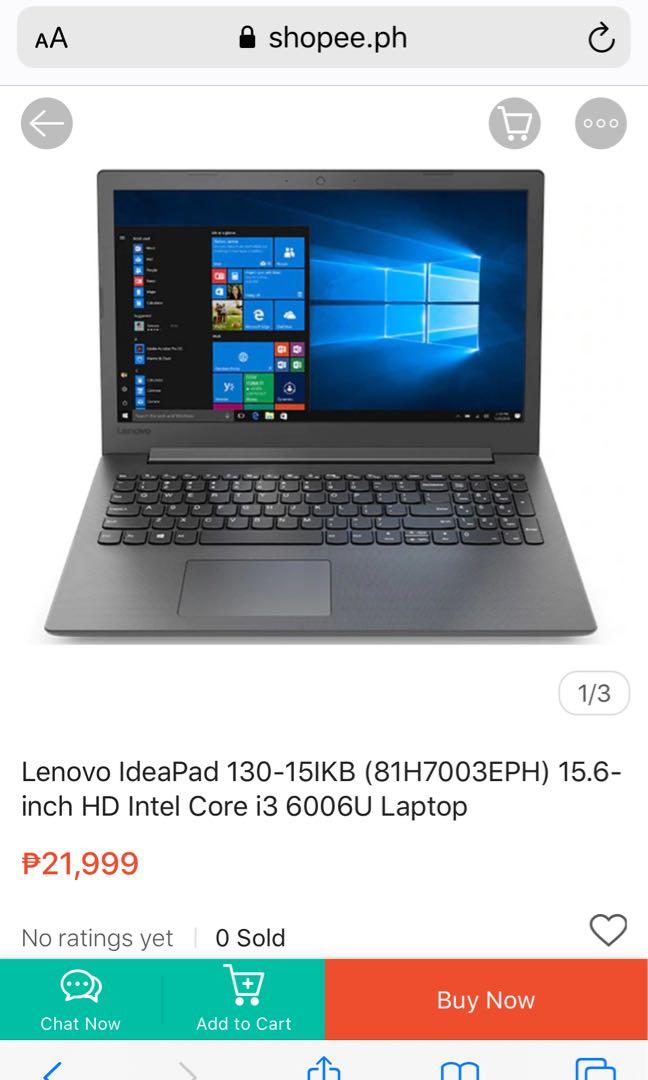This image depicts a product listing page on the website "shoppy.ph," showcasing a Lenovo IdeaPad 130-15iKB laptop, model number 81H7003EPH. The laptop features a 15.6-inch HD display and is powered by an Intel Core i3-606U processor. The listed price for the device is 21,999 pesos. The product has no ratings and has not yet been sold, as indicated by "0 of 0 have been sold." The image highlights multiple color options available for the laptop, including black, orange, and green. Additionally, the page includes actionable buttons such as "Chat Now," "Add to Cart," and "Buy Now" for customer convenience.